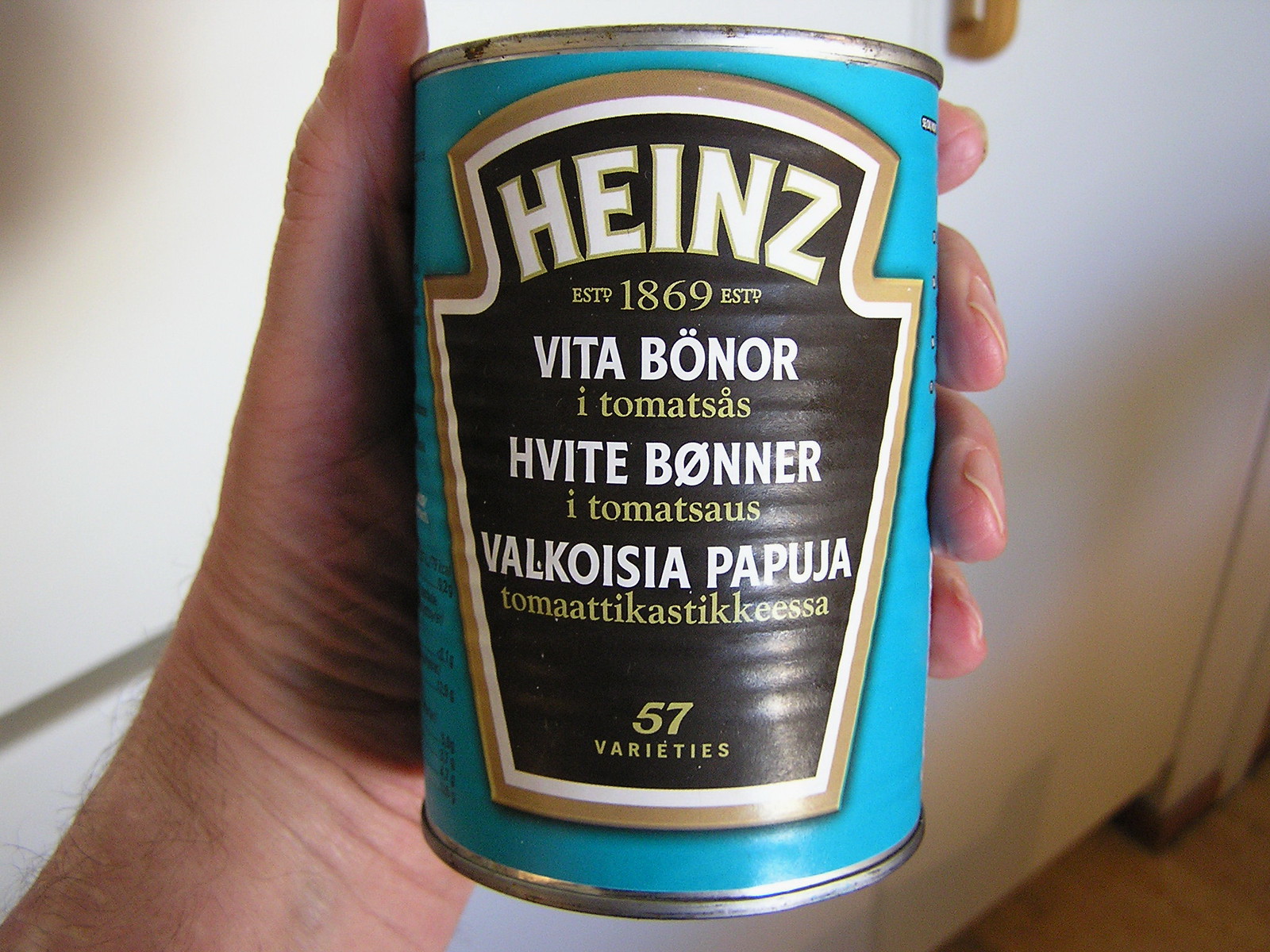An unusual can of Heinz tomatoes is featured, distinctively marked by its international labeling. The can prominently displays the iconic Heinz logo with "Established 1869," although it intriguingly spells 'Established' as "E-S-T-V." There are inscriptions in three different languages, adding to its eclectic nature. One of the languages appears to be Greek; another could potentially be from Spain, although the specific dialect is unclear. The third language is perplexingly foreign, not resembling Spanish or any other familiar script. This can, with its global linguistic tapestry, represents the diverse reach of Heinz products across different cultures and regions.